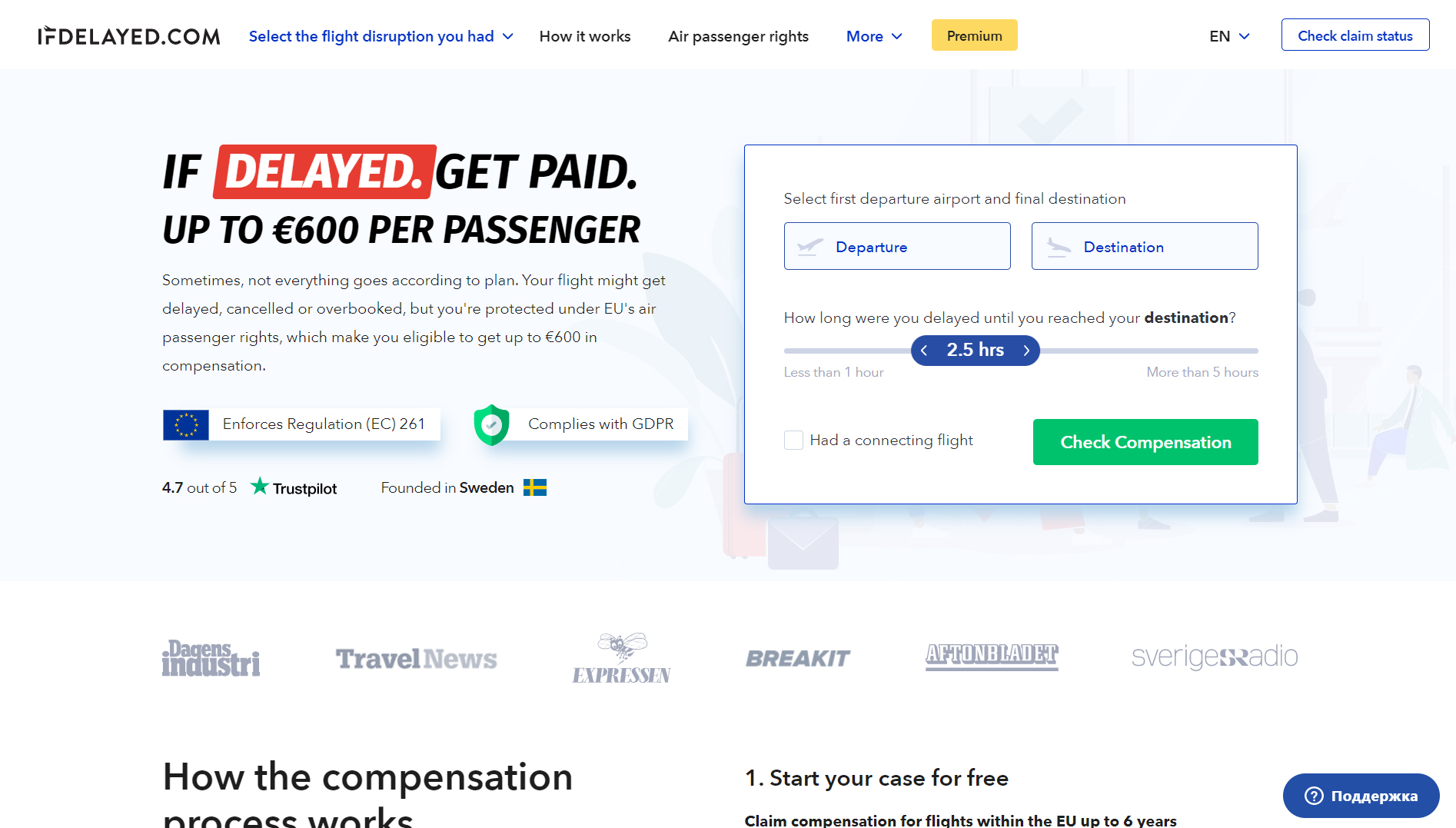The website ifdelayed.com offers a platform for passengers to claim compensation for flight disruptions. The homepage features a top navigation bar with options such as 'Select the Flight Disruption You Had,' 'How It Works,' 'Air Passenger Rights,' and 'More,' all aimed at guiding users through the claim process. A prominent yellow box labeled 'Premium' and a blue-outlined box with 'Check Claim Status' in blue letters are also visible in the top right corner, providing quick access to important features.

The main section of the page highlights the message: "If delayed, get paid up to 600 euros per passenger." This is presented with the word "delayed" in bold white letters on a red background, while the rest of the text is in black on a white background. The website explains that flight delays, cancellations, or overbookings can make passengers eligible for compensation under EU air passenger rights, up to 600 euros.

Two logos are featured underneath this information: one indicating enforcement of Regulation EC 261 with an image of the European Union flag, and another showing a shield with a green check mark, indicating GDPR compliance. Below these logos, a Trustpilot rating of 4.7 out of 5 stars is displayed, alongside the text "Founded in Sweden" with a Swedish flag.

On the right side of the homepage, there's an input box for users to enter their departure and destination airports, accompanied by a slider to adjust the delay duration, currently set at 2.5 hours. A green box labeled 'Check Compensation' is available for users to initiate the claim process. Logos of various travel news outlets are displayed further down the page, lending credibility to the site.

At the very bottom, the website explains the compensation process: 
1. Start your case for free.
2. Claim compensation for flights within the EU up to six years.
(Note: The description is cut off at this point.)

Overall, ifdelayed.com serves as an accessible and informative resource for air passengers seeking compensation for flight disruptions.